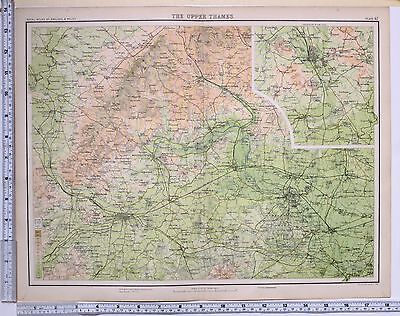This photograph depicts a detailed map titled "The Upper Thames," bordered by a thin black line and set against a faded yellowed parchment background. The map features a main color scheme of green, white, and shades of brown and pink. Dominating the lower right section of the map is a large green area, which transitions through white in the middle to an orangish-brown or pinkish hue in the upper part, with occasional green sections in the upper corners. An intricate network of black roads crisscrosses the map, heavily clustered in the bottom right region.

Two rulers provide a sense of scale for the map. One vertically aligns along the left-hand side, spanning from the bottom left to the top left corner. Due to the distance from the camera, the measurements on this ruler are not clearly discernible. The second ruler runs horizontally at the bottom of the map, extending from the bottom left to the bottom right. There's a small gap between these rulers, which intersect precisely at the bottom left corner of the map.

In addition, a white-outlined inset appears in the top right corner, offering a close-up view of a densely road-networked green section. The overall composition and framing of the photograph emphasize the scale and detailed topographical features of the map.